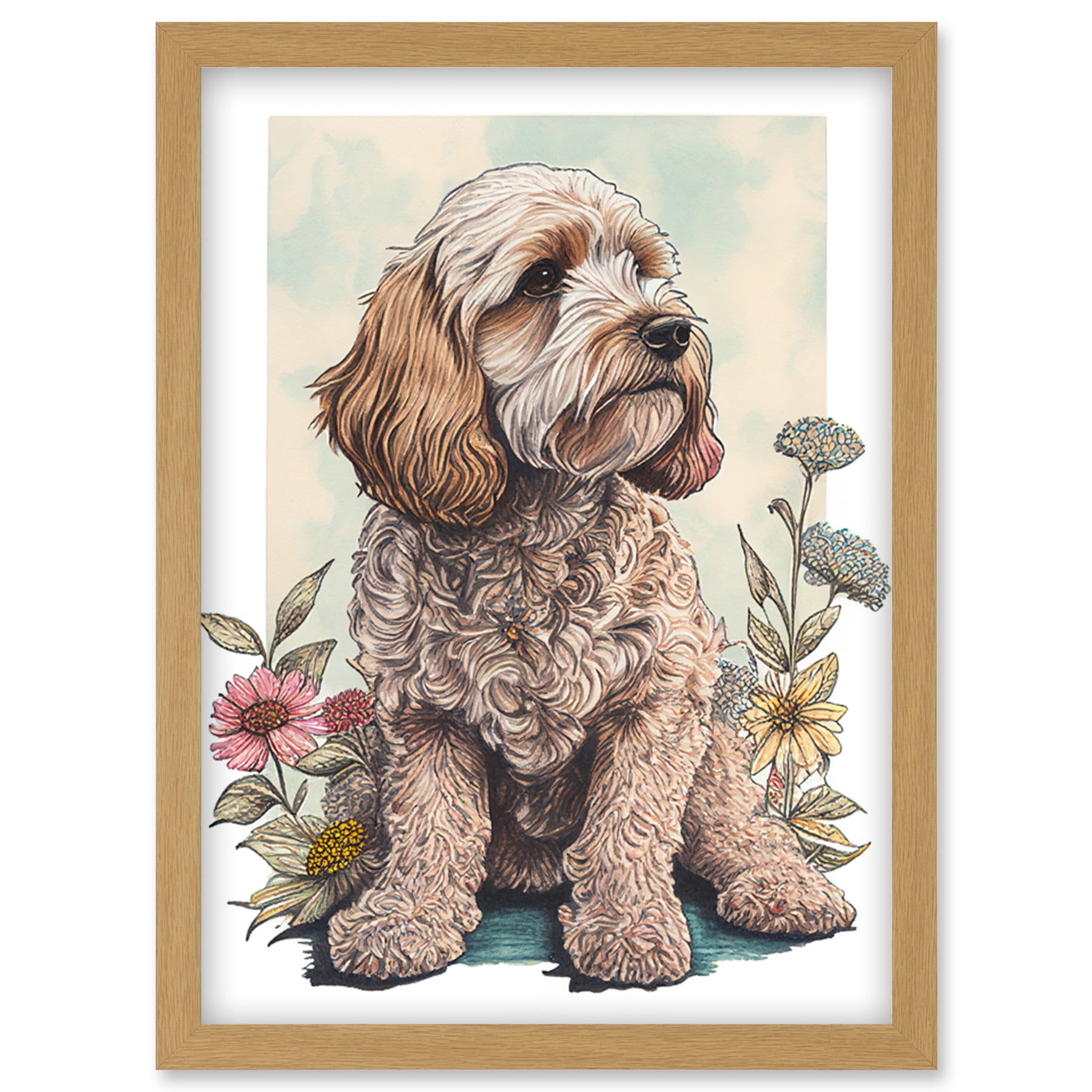This framed artwork showcases an adorable, fluffy puppy with curly, light brown fur that covers its entire body, including its paws, making them indistinguishable beneath the thick coat. The puppy's droopy ears are a darker brown, as are the areas around its eyes, nose, and bottom lip. The puppy gazes to the right, exuding a gentle, inquisitive expression. Surrounding the puppy are a variety of vibrant flowers—pink, yellow, and light blue blooms on the right and primarily pink and yellow flowers on the left, adding a lively floral backdrop. Beneath the puppy is a subtle depiction of a dark green or bluish-green area, possibly suggesting a small, reflective puddle of blue water. The entire image is elegantly enclosed in a simple yet classy wooden frame with a white border, enhancing the overall charm of this soft, endearing composition.